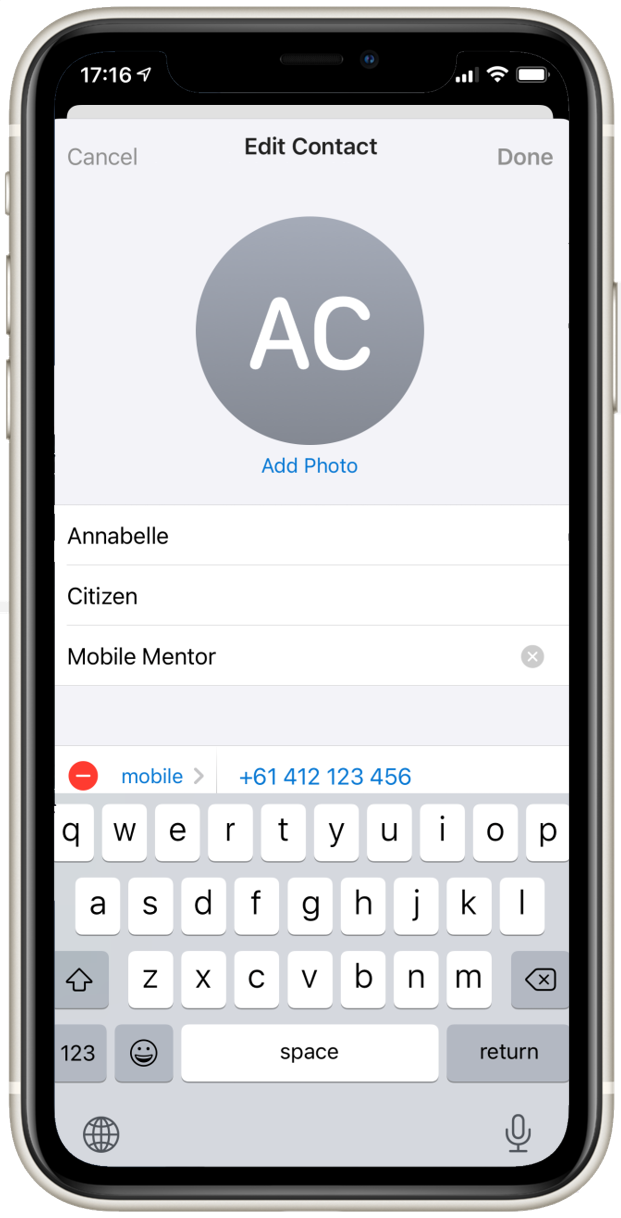The image displays a smartphone screen with the time set to 7:16. The interface shows an editing contact window. On the left, there's a "Cancel" button, and on the right, a "Done" button. A gray circle with the letters "AC" in white appears, surrounded by app icons in varying colors. Specifically, there's a blue "Photos" app icon, labeled "Annabelle - Citizen Mobile Mentor." To the right, there's another gray circle containing a white "X," and a red circle with a white dash. 

Further details reveal "Mobile" in blue text followed by a right arrow, and the contact number "+61 412 123 456" also in blue. The keyboard interface features an up arrow, a house icon turned left with an "X," and numeric keys "1," "2," "3." Below the numbers are a smiley face key, a spacebar, and a return key. At the bottom of the keyboard, there is a globe icon on the left and a microphone icon on the right.